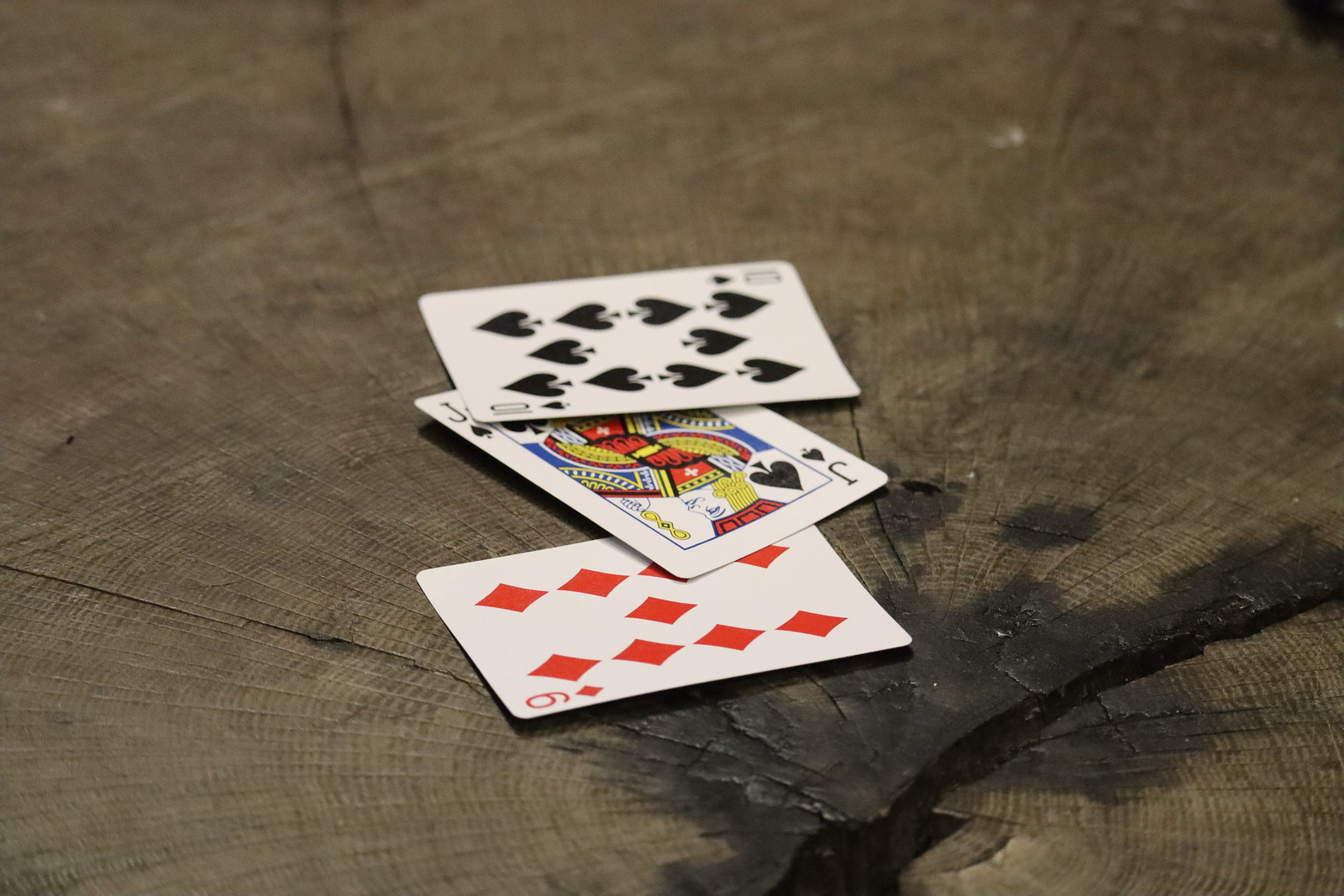The image showcases a rustic tabletop crafted from a tree trunk sliced in half, displaying a prominent deep crack running through its center. The wood's natural rings are vividly visible, adding rich texture to the piece. Dark stains accentuate the crack, providing a striking contrast against the wood's grain. Three playing cards are meticulously placed on the surface: the 10 of Spades, the Jack of Spades, and the 9 of Diamonds. The photograph has a subdued lighting environment, lacking any specific light source, which lends a soft, ambient quality to the composition. The edges of the image and the top part of the 10 of Spades card appear slightly blurred, focusing the viewer's attention on the central elements. Despite the minimalistic setup, the high-quality resolution suggests it was taken with a sophisticated camera, likely a high-end smartphone.